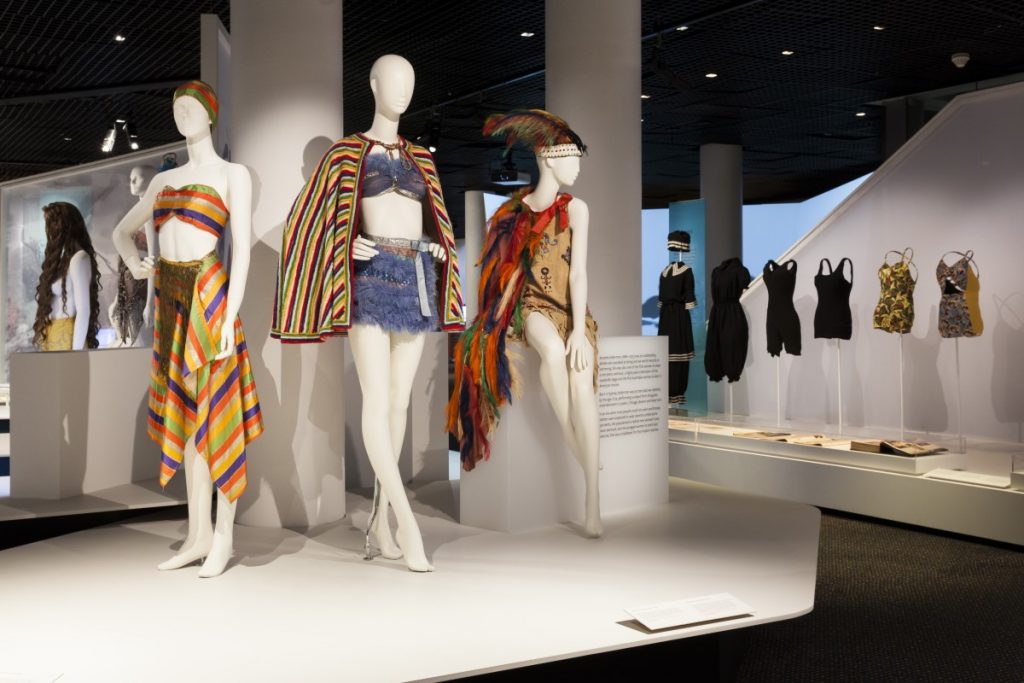The image portrays an elaborate fashion display in what appears to be a museum or high-end department store. At the forefront, three mannequins stand in a row on a platform, each adorned in distinctive summer or beachwear ensembles. The left mannequin wears a colorful striped outfit, consisting of a bra top, a flowing skirt with stripes in orange, yellow, green, purple, and tan, and a matching head wrap. The central mannequin showcases a feathery-textured ensemble, featuring a short skirt and a bra top in cool hues, accented by a silver belt, and topped with a vibrant striped cape. The right mannequin dons a tan dress with a whimsical feathery cape draped over her shoulder, boasting feathers in purple, orange, and green, along with a matching headdress. Flanking the platform on the right side, a series of bathing suits from various eras are displayed, including a black bloomer-style suit from the 1920s and progressively less covering one-piece suits. These historic bathing attires are complemented by accompanying descriptive text blocks and open books, providing informative context to the exhibit.